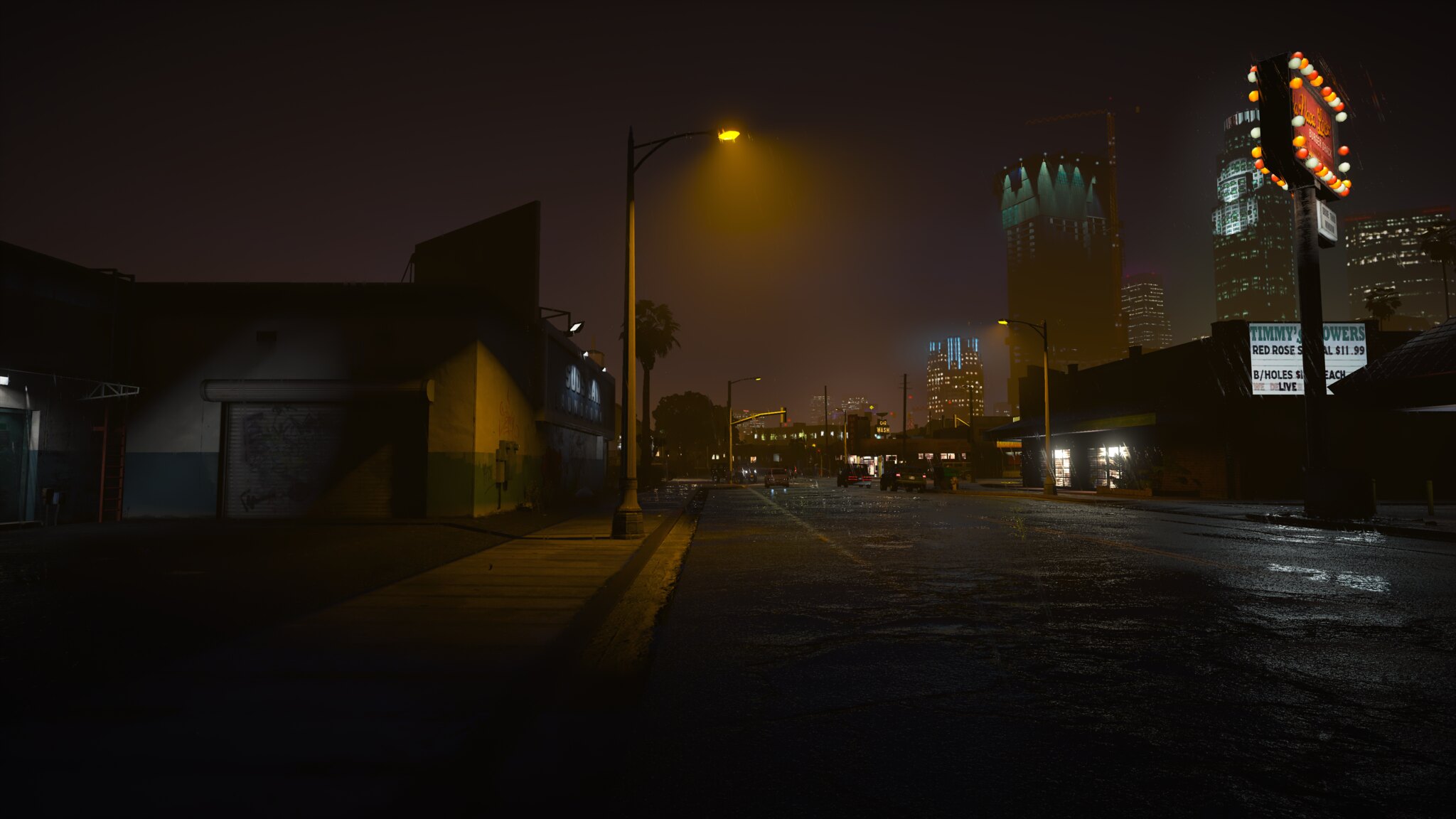This digital image, created by AI, presents an extraordinarily lifelike rendering of a city street at night. The scene is bathed in darkness, with a warm, glowing street lamp providing a comforting contrast. Across the street, a marquee sign announces a "Red Rose Special" for $11.99, while another sign illuminates the area with its vibrant neon style. In the background, towering skyscrapers with lit windows contribute to the urban atmosphere. The street, slick and glistening from the rainfall, mirrors the lights from the city and the lampposts, enhancing the scene with reflective raindrop splashes that add an element of realism and depth.